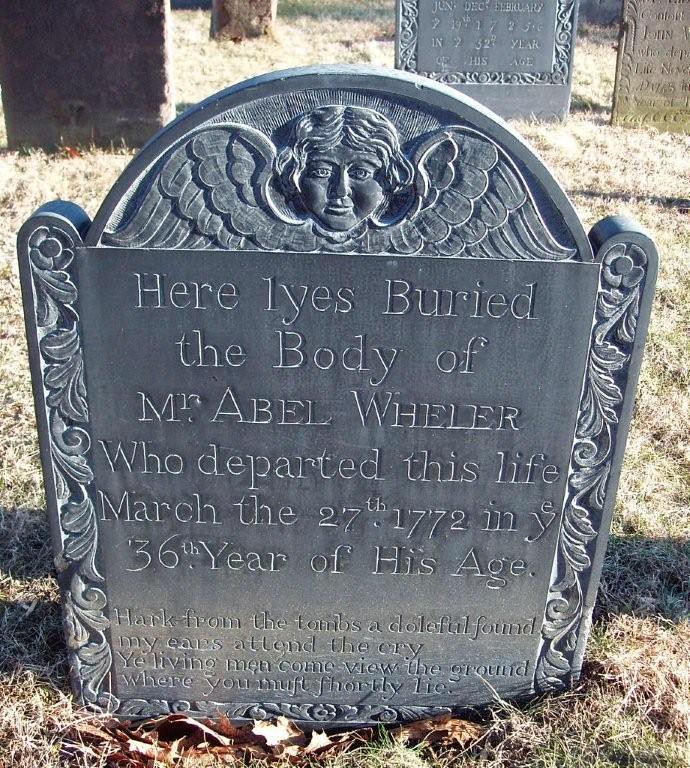In the foreground of this serene yet somber image, we see an aged gravestone standing slightly crooked in a seemingly forgotten cemetery. The gravestone, made of gray slate and weathered by time, features a beautifully carved angel at the rounded top, symbolizing protection and peace for the departed. Floral wreaths with intricate scrolls and vines embellish the sides, adding a touch of elegance to the somber stone. 

The inscription reads: "Here lies buried the body of Mr. Abel Wheeler, who departed this life March the 27th, 1772, in ye 36th year of his age. Hark from the tombs a doleful sound; my ear attends the cry: Ye living men, come view the ground where you must shortly lie." Though parts of the text are worn and difficult to decipher, the poignant message remains clear.

In the background, four other gravestones, equally ancient and worn, stand in silent witness amidst a patchy, brown lawn with very little green grass visible, further emphasizing the passage of time in this sacred place. The scene captures a poignant moment in history, a testament to lives once lived and the enduring peace of the cemetery.